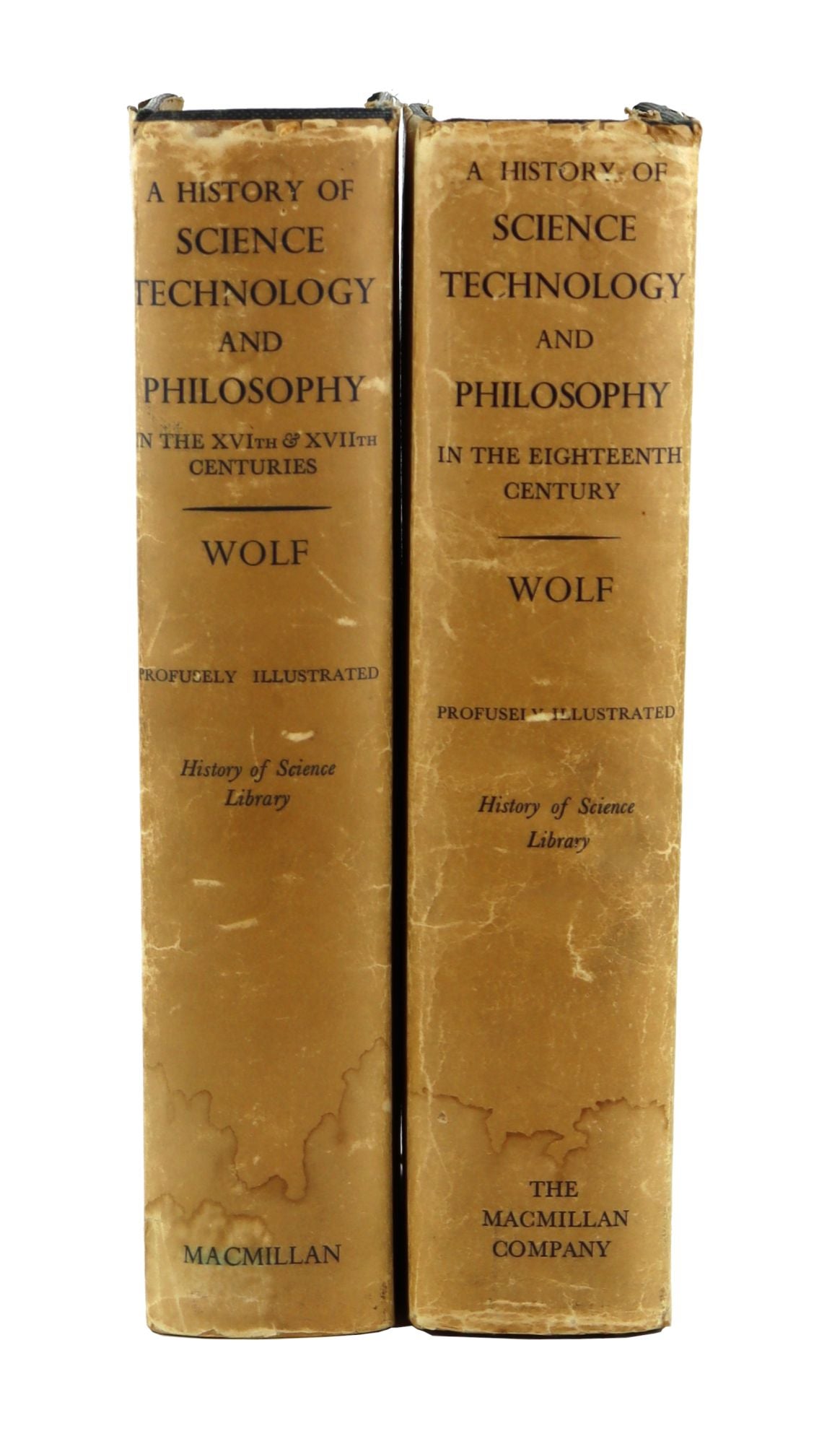The photograph shows the spines of two worn and possibly water-damaged textbooks side by side, set against a plain white background, likely taken in a light box. Both books are of a light tan-beige color and exhibit significant signs of aging, with crinkled covers and some text on the spines rendered unreadable due to surface damage. The book on the left is titled "A History of Science, Technology and Philosophy" and features additional text noting it is a part of "A History of Science Library," published by Macmillan and authored by Wolff. The book on the right, similar in appearance and condition, is titled "A History of Science, Technology and Philosophy in the 18th Century," also by Wolff, marked as a part of the same series and published by The Macmillan Company. Both books are described as "profusely illustrated," highlighting their comprehensive nature.